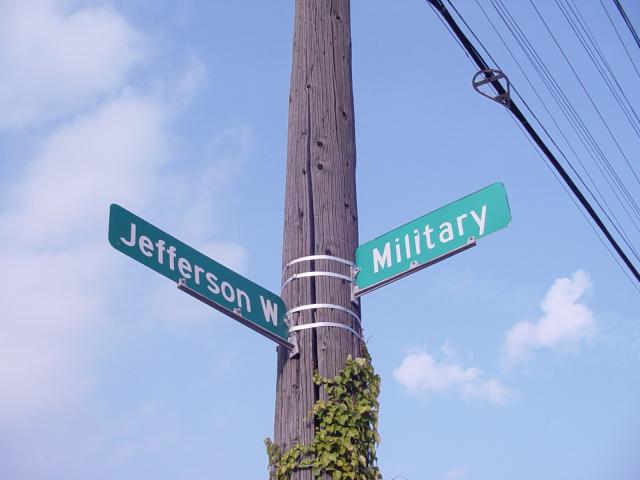The image captures an upward view from the ground of a brown wooden utility pole bordered by bright green leafy ivy at its base. Affixed to the post with light gray metallic ties, two street signs extend outward in opposite directions. The shiny, reflective signs are green with white text; the left sign reads "Jefferson W," and the right sign reads "Military." In the clear blue sky background, wisps of fluffy white clouds float, while several black power lines appear in the upper right corner, adding an element of urban infrastructure to the serene setting. The quality of the image conveys a slightly vintage feel, suggesting it might have been taken with an older camera.